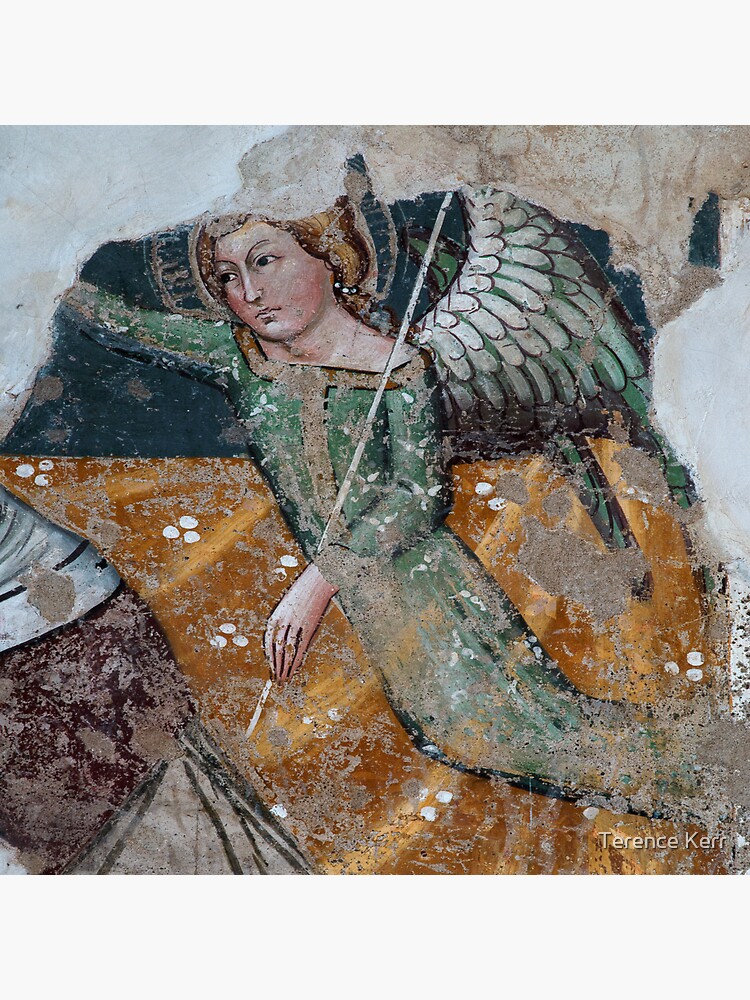The image is a square detail of a weathered, medieval-period fresco, possibly part of a larger mural akin to those in the Sistine Chapel. The artwork, which appears to be painted on a marble surface, features an angelic figure with white yet gradually darkening to gray wings. The angel, depicted with blonde braided hair and pink cheeks, has a neutral or slightly sad expression. She wears a flowing green dress adorned with golden accents, particularly around the collar and button area, and her right arm extends outward, cut off just below the elbow, while her other hand holds a rod. A faint halo encircles her head, and her feet are off the ground, suggesting she is flying. The background includes rich greens, golds, browns, whites, and grays with various accents and dots. The fresco shows signs of age and damage, with chipped paint at the top. In the lower right corner, there is a watermark in small white lettering that reads "Terrence Kerr."